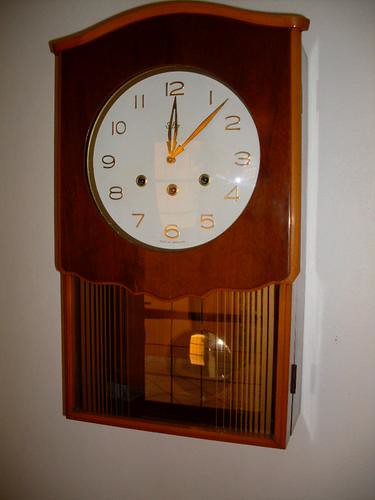The indoor photograph captures a beautifully crafted, wall-mounted wooden clock against a white wall. The clock shows the time as 12:07 with gold-colored hour and minute hands. Its round face, which is white, features gold numbers and includes three small dark circles near the center. The clock’s rectangular wooden frame is finished in two shades of brown, giving it a polished, brand-new appearance. Below the clock dial, encased in glass, a golden pendulum can be seen, adding an elegant touch to the timepiece. A slight reflection of the camera flash is visible to the right of the clock. Despite being well-lit, the lower part of the clock appears a bit out of focus. The overall image is a slightly angled view, providing a detailed look at the intricate design and craftsmanship of the clock.